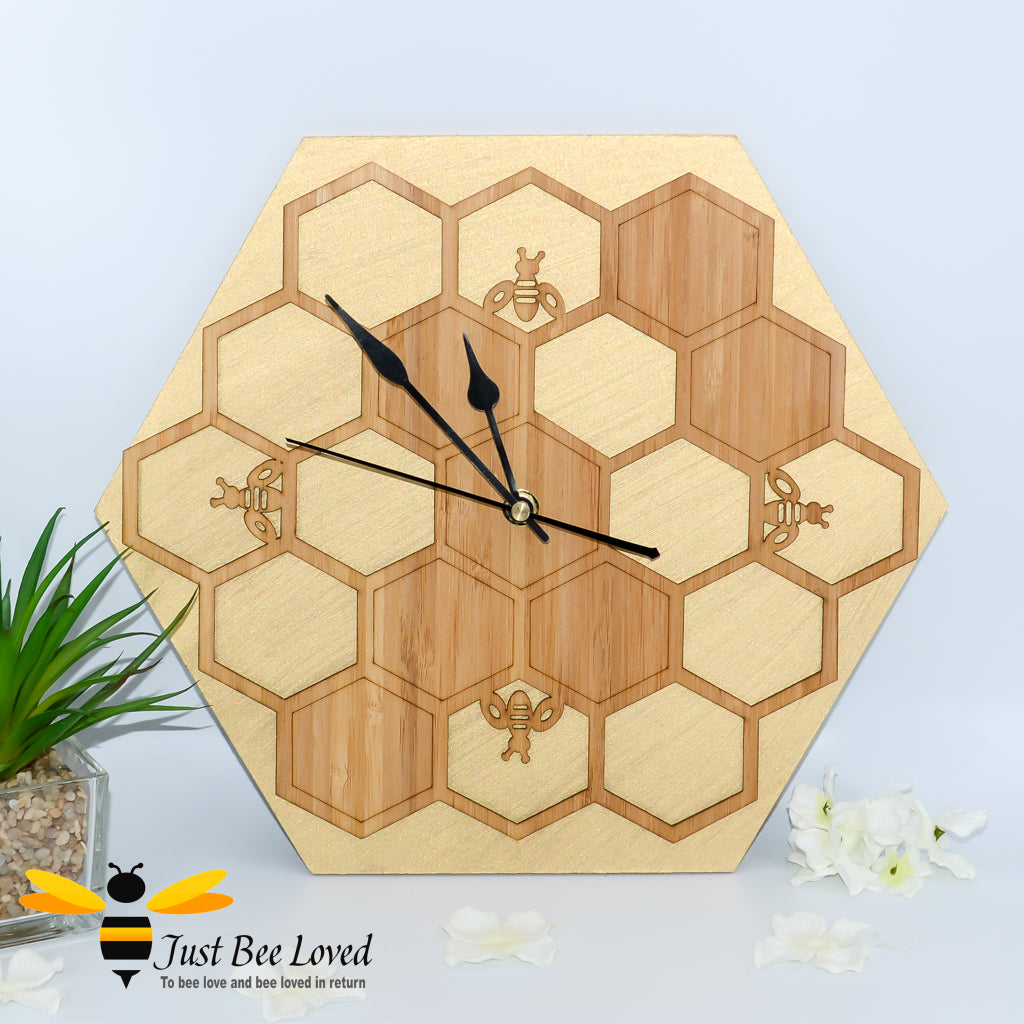The image features a hexagonal clock crafted from light blonde wood. At the center, there is a detailed illustration of a beehive, rendered in a darker brown shade. Selected honeycombs within the beehive are shaded for depth and texture. At the positions corresponding to 12, 3, 6, and 9 on the clock face, small brown bees are depicted. These bees have black bodies with tiny white stripes. The clock's hands, including the hour, minute, and a very thin second hand, are all in black.

The background of the scene is a soft light blue, and the clock sits upon a similarly colored base. To the right of the clock, there are white petal-like flower embellishments. In front of the clock sits a clear planter filled with small rocks and green leafy plants.

At the bottom of the clock, a label reads "Just Bee Loved," where "Bee" is cleverly illustrated as a bee. The bee on the label has a black head, two small black antennas, yellow wings on each side, and a body striped with black and yellow. Below this whimsical bee illustration, the phrase "Be loved and be loved in return" is inscribed, further enhancing the theme of love and nature.